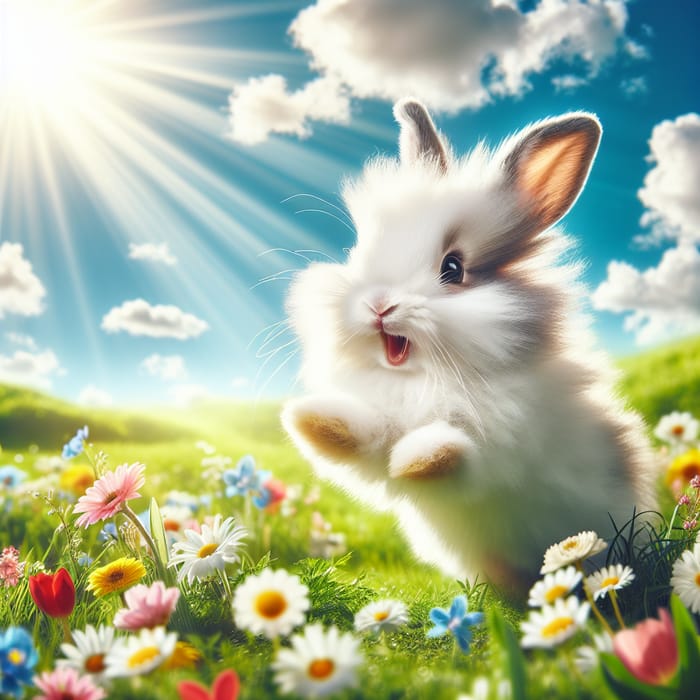The image is a computer-generated depiction of a very fluffy white bunny mid-jump in a lush prairie field. The bunny, which has one visible dark eye and a half-smiling, open mouth, appears to be launching itself with its hind feet while both of its front paws are raised in the air. The bunny's fur is soft and slightly gray around the face. The field is vibrant with a mix of flowers, including white and yellow daisies, red tulips, blue flowers, pink daisies, and yellow dandelions. In the background, rolling hills meet a light blue sky filled with fluffy cumulus clouds. Sunlight, depicted as a clear white projection, streams down from the top left corner, illuminating the bunny and the colorful field in what seems to be a serene, springtime scene, possibly themed around Easter.